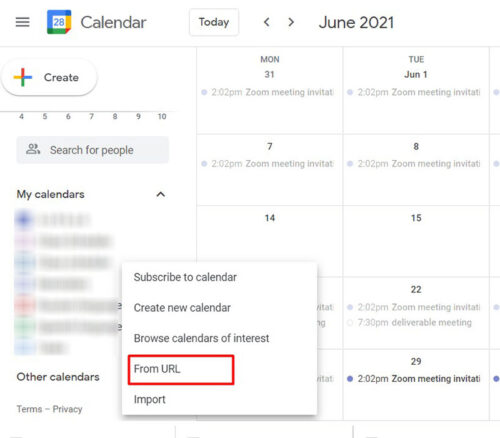The image displays a Google Calendar interface from June 2021, highlighting the feature to add new calendars. The top bar features familiar navigation elements: a hamburger menu icon on the left, a 'Today' button, directional arrows to move forward and backward in the calendar, and the current month and year, June 2021, displayed prominently. 

On the left-hand side, below the Google Calendar logo, there is a 'Create' button with a plus sign, a 'Search for people' button, and sections labeled 'My calendars' and 'Other calendars'. The main calendar area on the right shows individual days as small boxes with scheduled meetings marked within them.

The focal point of the image is a dropdown menu for adding a new calendar, which includes options such as 'Subscribe to calendar,' 'Create new calendar,' 'Browse calendars of interest,' 'From URL,' and 'Import.' A red box highlights the 'From URL' option, indicating its importance in this context. Additionally, a small section at the bottom of the page links to terms and privacy policies.